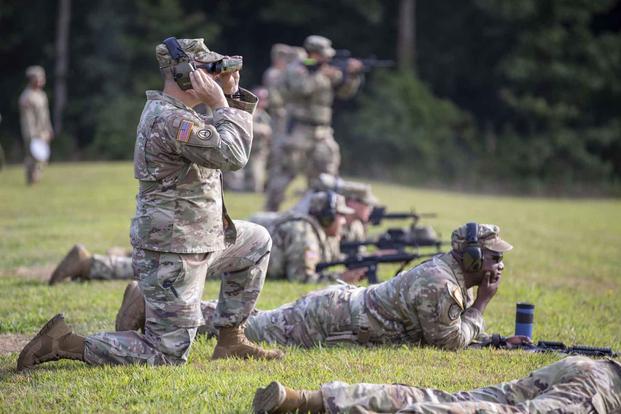The image captures a group of military personnel in a training session, all dressed in camouflage fatigues and brown boots, set against a backdrop of green trees. The soldiers are arranged in a staggered line facing the right, with some lying prone on a grassy field and others kneeling or standing. The men on the ground have their rifles aimed forward, supported by the earth. Among them, a black soldier props his chin on his hand next to a blue thermos mug. Nearby, a kneeling soldier with a pair of binoculars, wearing ear protection and a cap with an American flag patch, appears to be observing the target area. In the far background, slightly out of focus, more soldiers stand with their rifles aimed, with one standing figure on the upper left holding a white square object, possibly paperwork. All soldiers are equipped with noise-canceling earmuffs to protect against gunfire noise, creating a scene indicative of a focused training exercise.